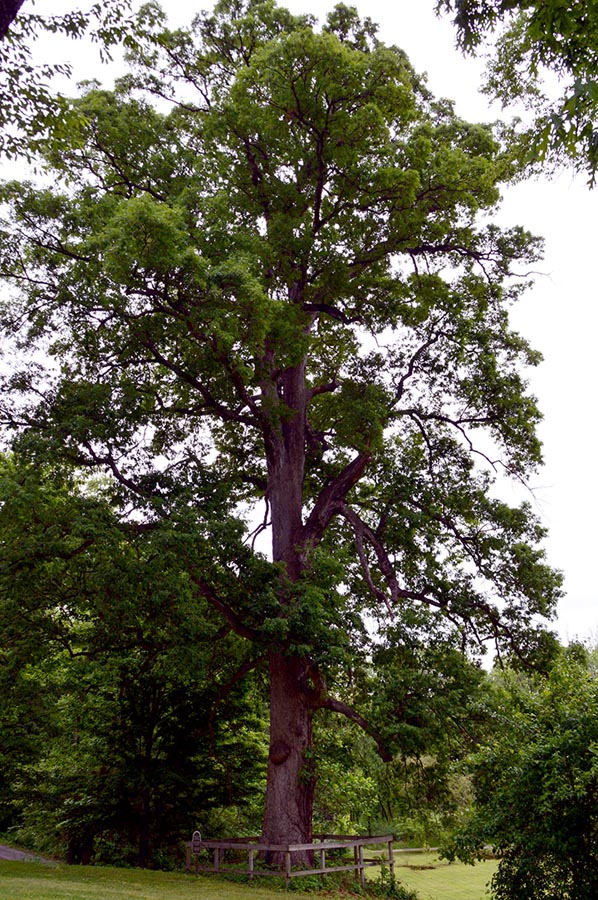This photograph captures a remarkably tall, prominent tree situated in a park or wooded area, distinguished by its extensive height and lush green foliage. The tree’s substantial brown trunk, which exhibits a faint purplish hue likely due to the overexposed, completely white sky, extends majestically from the bottom to the top of the frame. Encircling the tree at its base is a square wooden fence, designed to protect and possibly highlight its importance. Within this fenced area, ivy or other greenery intertwines around the trunk. The tree is surrounded by shorter trees, contributing to a vibrant, green landscape. Additionally, there is a small brown sign mounted to the left of the fence, though its inscription remains unreadable. The image conveys the tree's grandeur and the serene environment it inhabits.